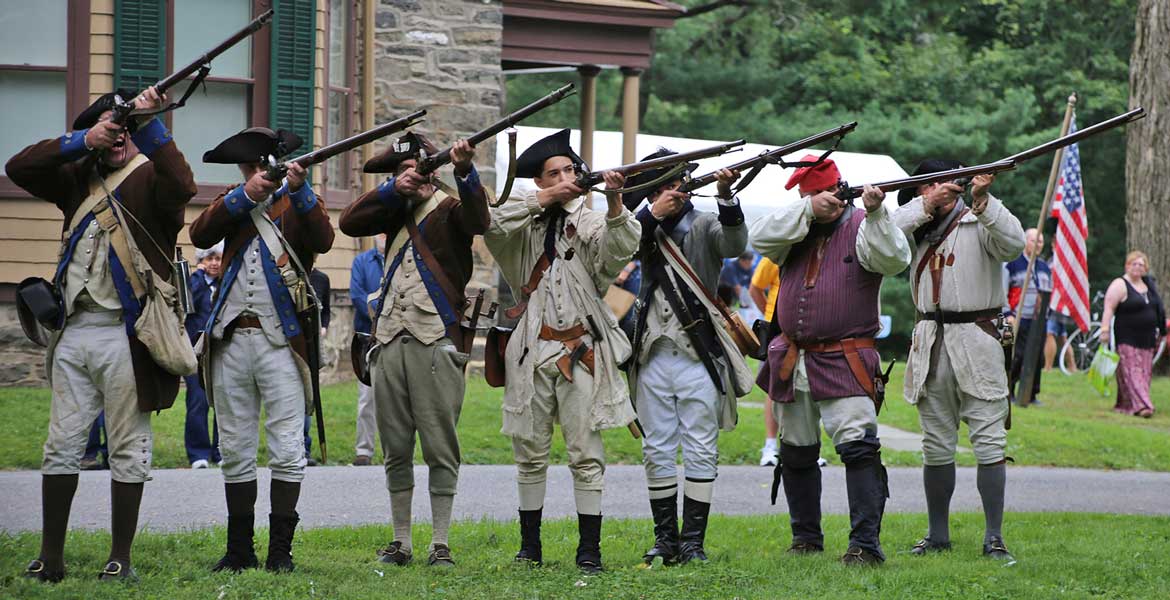In this detailed, outdoor daytime photograph, a group of seven reenactors dressed as colonial Minutemen or militia form a line facing the camera, performing a mock setup where they are about to fire their long-barreled rifles. These reenactors are adorned in traditional colonial attire, featuring black boots, beige or occasionally dark green trousers, blue colonial long coats, and a mix of black tricorn hats and a single red bandana. Each man has a bag slung across his body, with two of them sporting fanny packs. The rifles, uniformly brown, are held close to their heads with barrels slightly elevated and pointing to the right. In the background, an old colonial building is visible on the left, while modern-day onlookers stand on the right, attending what appears to be a historical celebration or festival. An American flag stands prominently in the upper right quadrant of the image. The setting includes a street—either cement or gravel—flanked by grass where the reenactors are positioned.